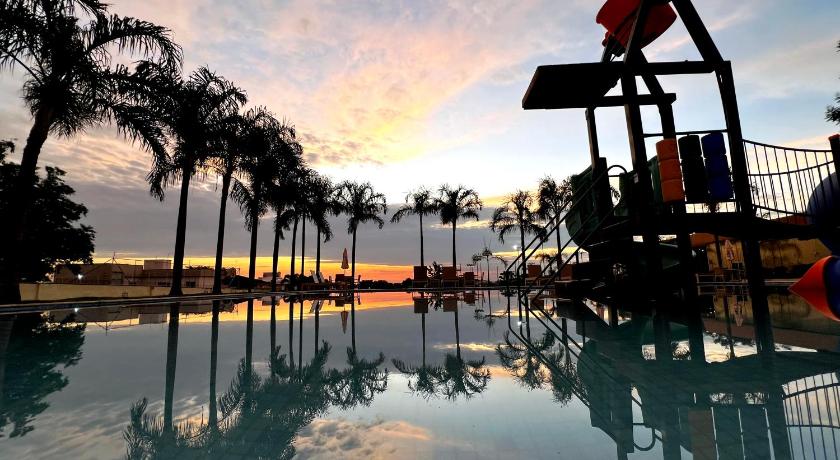This image captures a serene water park scene at sundown. The sky transitions from a light blue with white and yellow clouds to a grey section in the middle, ultimately showcasing a beautiful orange and yellow horizon near the ground. The water park features a large, calm pool, surrounded by several dark, silhouetted palm and pine trees. The pool's mirror-like surface reflects the vibrant sky and foliage, adding to the tranquility of the scene. On the left and right sides of the pool, there are platforms with slides and stairs descending into the water. The scene also includes various structures such as a play area, swing set, ladders, and foam dividers. A few lawn chairs and beach umbrellas are scattered around the pool, hinting at a resort-like environment. The overall atmosphere is peaceful and reflective, with the colors of the setting sun beautifully enhancing the entire view.